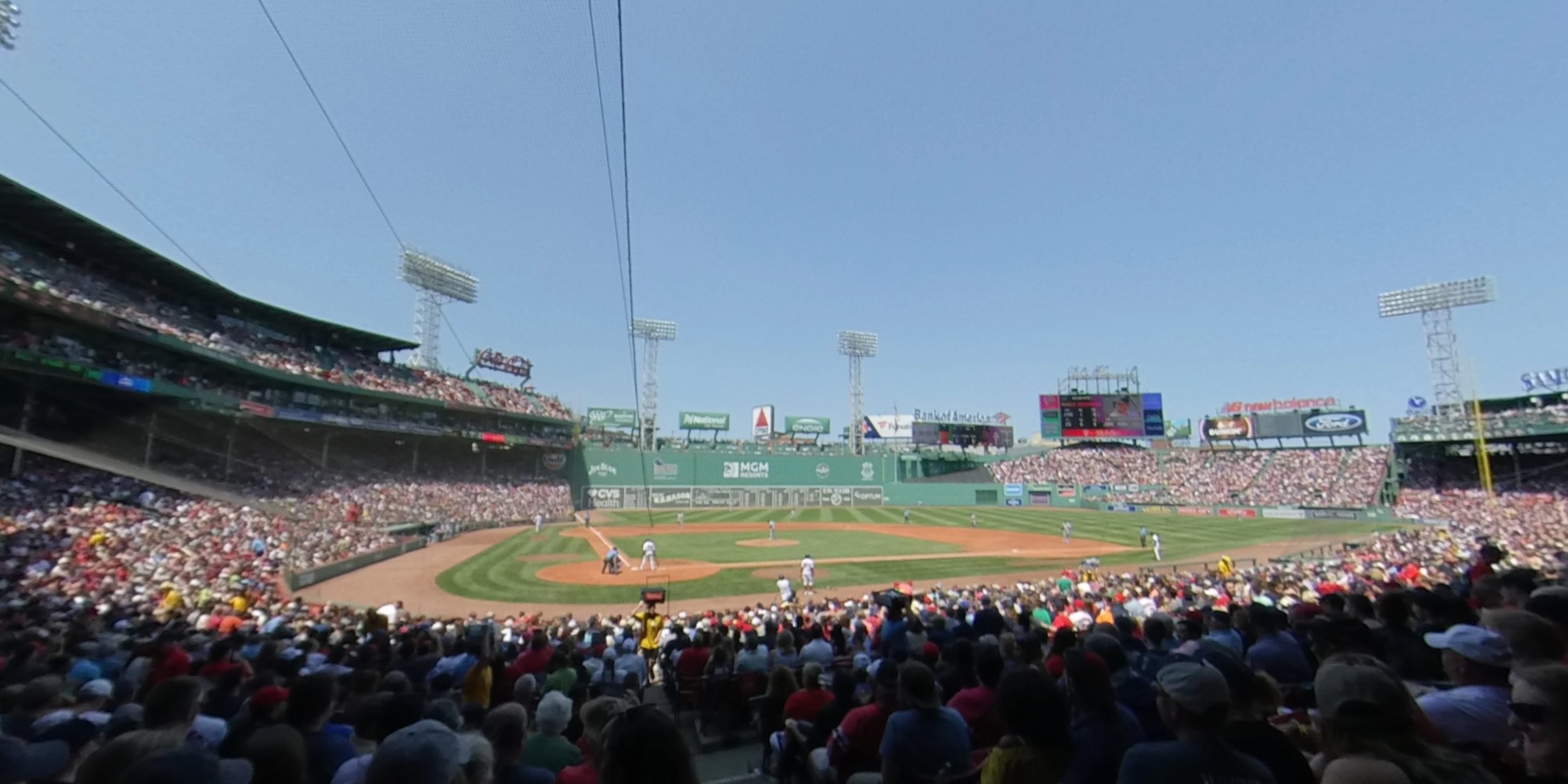This image, taken from about 20 rows back and slightly to the right behind home plate, captures the vibrant atmosphere of a daytime baseball game in a large, three-story stadium filled with spectators. The clear, blue sky above enhances the vivid colors in the scene: the lush green of the baseball field, the orange dirt of the diamond, and the multitude of shirts worn by fans, ranging from red and blue to yellow. Many of the spectators, numbering over a thousand, are sporting white hats, though they appear as a blur of heads in the packed stands. 

The baseball players on the field are clad in white uniforms, distinguishable from the crowd. Surrounding the field are various billboards and advertisements, including prominent ones for Ford and Bank of America, and another featuring a red triangle. Additionally, a jack-o-lantern ad can be seen, along with green billboards. In the back right, a scoreboard displays a picture of a player and another Ford advertisement. Four horizontal banks of headlights, each containing around 100 lights, illuminate the field, emphasizing the vastness and the lively energy of the stadium.